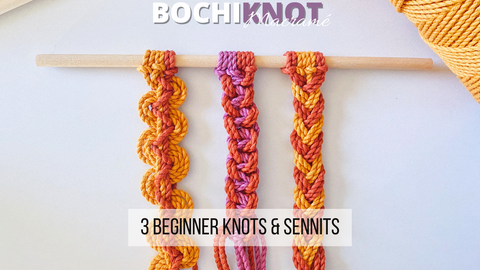The image appears to be a screenshot or thumbnail from a video, as indicated by various captions and their elements. At the top of the image, the text reads "Bocci Knot", with "Bocci" in white and "Knot" in purple. Below this header, there is an additional cursive element in white, seemingly reading "Masure", superimposed over the purple text. The image highlights "Three Beginner Knots and Sentence" in black text against a semi-transparent white rectangle at the bottom.

In the background, a thin wooden rod is visible, with three distinct columns of crochet designs hanging from it. The knots are crafted from differently colored yarns, showcasing various knotting and braiding styles. The first column, located on the left, features yarns in yellow and red tones woven into a serpentine or S-shaped pattern. The center column consists of a mix of purple and red yarns, exhibiting a more intricate knotting style. The rightmost column once again uses yellow and orange yarns, resembling a Windsor knot. Additionally, there is a large ball of yarn situated in the top right corner of the image, reinforcing the crafting theme.